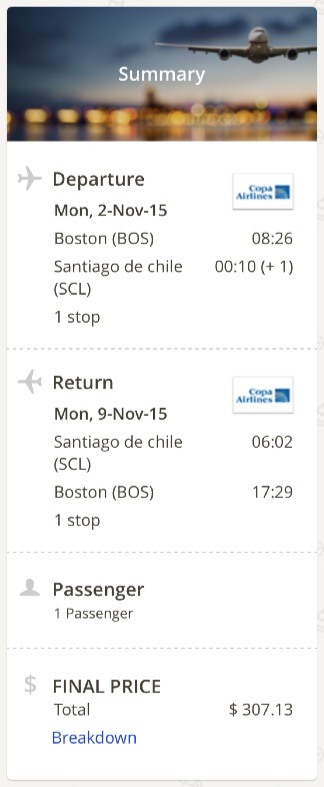A vertical, rectangular screenshot displays a flight itinerary, presumably captured from a mobile phone. At the top of the screenshot, a small photograph of an airplane in flight is visible. The background features a cityscape and a blurry sky. Overlaying this image, the word "Summary" is prominently displayed in white text.

Beneath the photo, a white background with black text details the flight information. Clearly marked, the Copa Airlines logo signifies the carrier. 

The itinerary lists a departure on Monday, November 2, 2015, from Boston to Santiago de Chile at 8:26 a.m., with one stop en route. The return flight is scheduled for Monday, November 9, 2015, departing from Santiago de Chile at 6:02 a.m. and arriving in Boston at 5:29 p.m.

The document confirms there is one passenger. At the bottom of the screenshot, the final price is clearly stated as $307.13. A clickable option, colored blue and labeled "Breakdown," offers further details on the pricing.